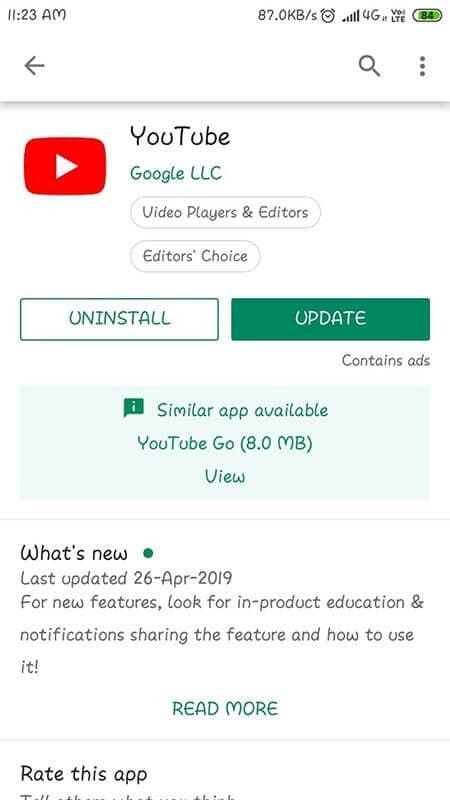The image displays a smartphone screen at 11:23 AM with the following details:

- **Memory Usage**: 87.0 kilobytes
- **Icons**: An alarm clock, full signal bars, and a battery level at 94%
- **Navigation**: A magnifying glass icon and a three-line menu icon on the right
- **App Details for YouTube**:
  - **Icon**: The familiar red square with a white play triangle
  - **Text**: "YouTube" in black, "Google LLC" in green
  - **Category**: Video Players and Editors
  - **Editor's Choice**: Highlighted in black with white text
  - **Options**: "Uninstall" or "Update" with "Update" highlighted
  - **Similar App**: "YouTube Go - 8.0 MB" with a view link
  - **Ads**: Indicates the app contains ads
  - **What's New Section**: Displaying a green dot, last updated on April 26, 2019
    - **Description**: For new features, look for in-product education and notification sharing
    - **Additional Info**: "Read more" option in green
- **Rate This App**: Section in black

The screen prompts the user to update the app with an `Update` button and allows rating the app based on user experience.